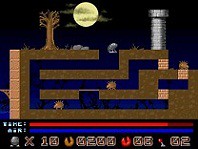This image is a detailed screenshot from an old-fashioned 8-bit video game, reminiscent of titles from the 90s or early 2000s. The scene features a maze constructed of brown bricks, which spans across the middle of the screen. Above the maze, a dark, nighttime sky serves as the backdrop, dominated by a large moon partially obscured by drifting grayish clouds. To the left of the moon stands a solitary brown tree, while on the right, a metal-tubed chute ascends, resembling a castle pillar or a structural element. The bottom of the image displays player information and game indicators: a red bar with white lettering nearly spans across the screen, followed by a blue bar, also with white text, extending all the way across. Additionally, mixed in with brown and jagged blue elements, there are numerous vague, gold and black images, intertwined with red, which likely represent progress or status indicators within the game.